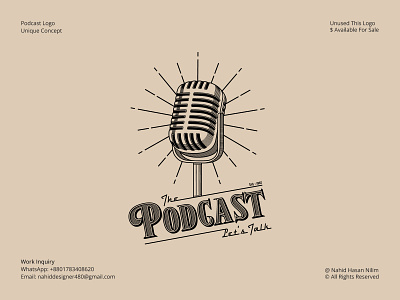The image is an advertisement, likely promoting a podcast or the possibility to advertise your own podcast. The central focus is a vintage, black-and-white depiction of an old-fashioned, boxy microphone, reminiscent of those placed on a stage stand. Below the microphone, the placeholder text "The [Blank] Podcast, Let's Talk" appears, suggesting that viewers can insert their own podcast name for advertising purposes. The phrase "The Podcast" is in a normal font, while "Let's Talk" is in cursive.

In the corners of the beige-toned poster are various details written in black text. In the upper left corner, it states "Podcast Logo, Unique Concept." The upper right corner reads "Unused, This Logo Available for Sale." The bottom left corner provides "Work Inquiry" information, including a WhatsApp number and an email address, though these details are hard to read due to their small font size. The bottom right corner bears a company name that's difficult to discern, followed by "All Rights Reserved."

Overall, the poster combines a nostalgic visual with practical information, offering a customizable advertisement platform for podcasts.